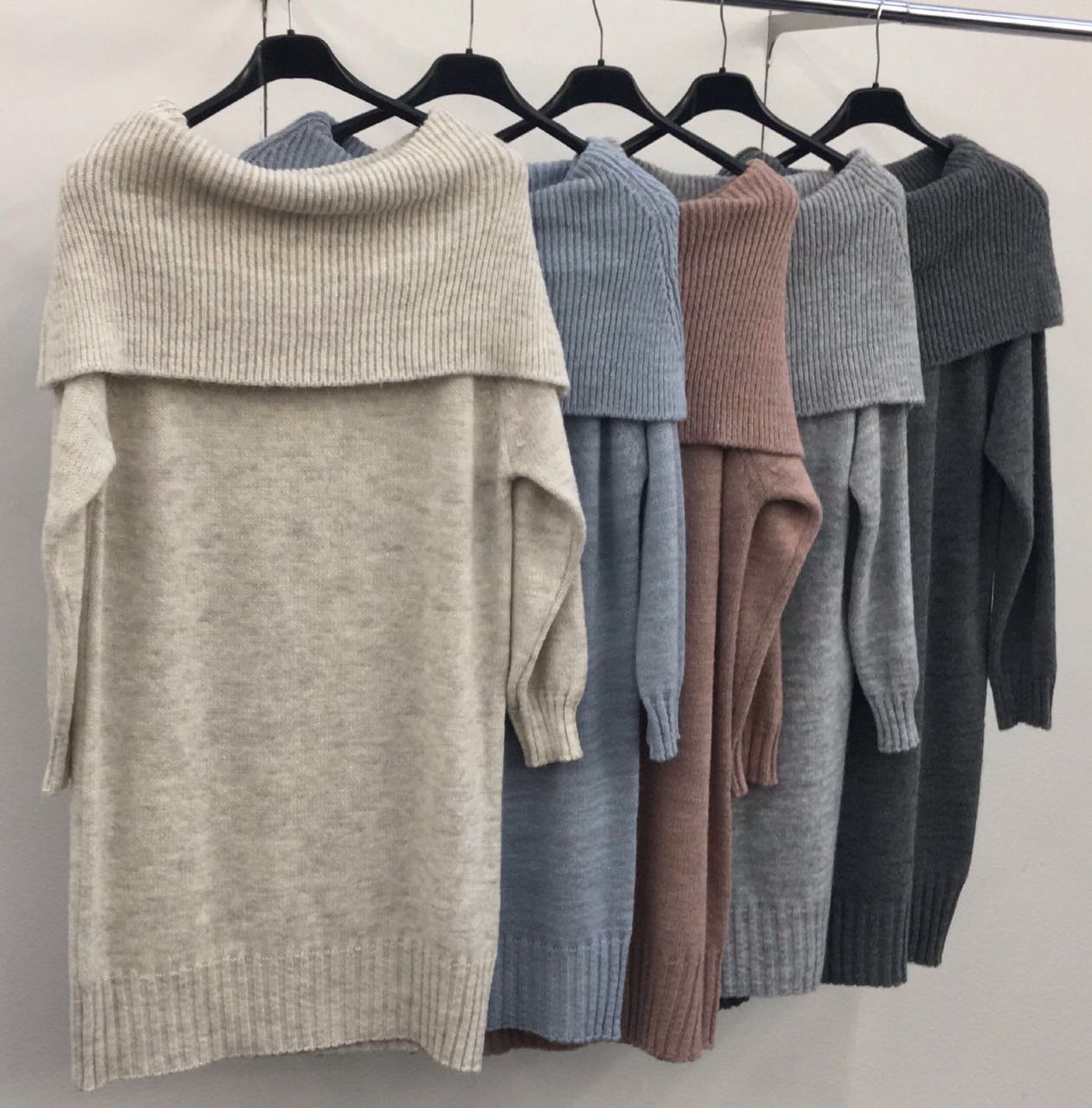This image displays five women's sweaters hanging on black hangers from a metal rod against a beige wall, reminiscent of a department store setup. Each sweater features a three-quarter length sleeve, a folded-over collar extending over the shoulders, and a band with vertical lines at the bottom. The material appears to be a cotton blend. The sweaters are identical in style but come in varying colors: the first on the left is a stone or light gray, followed by a periwinkle blue-gray, then a mauve brown, next a medium gray, and finally a deeper charcoal gray that’s almost black. Each hanger has a silver thin hook, contributing to the uniformity of the display.